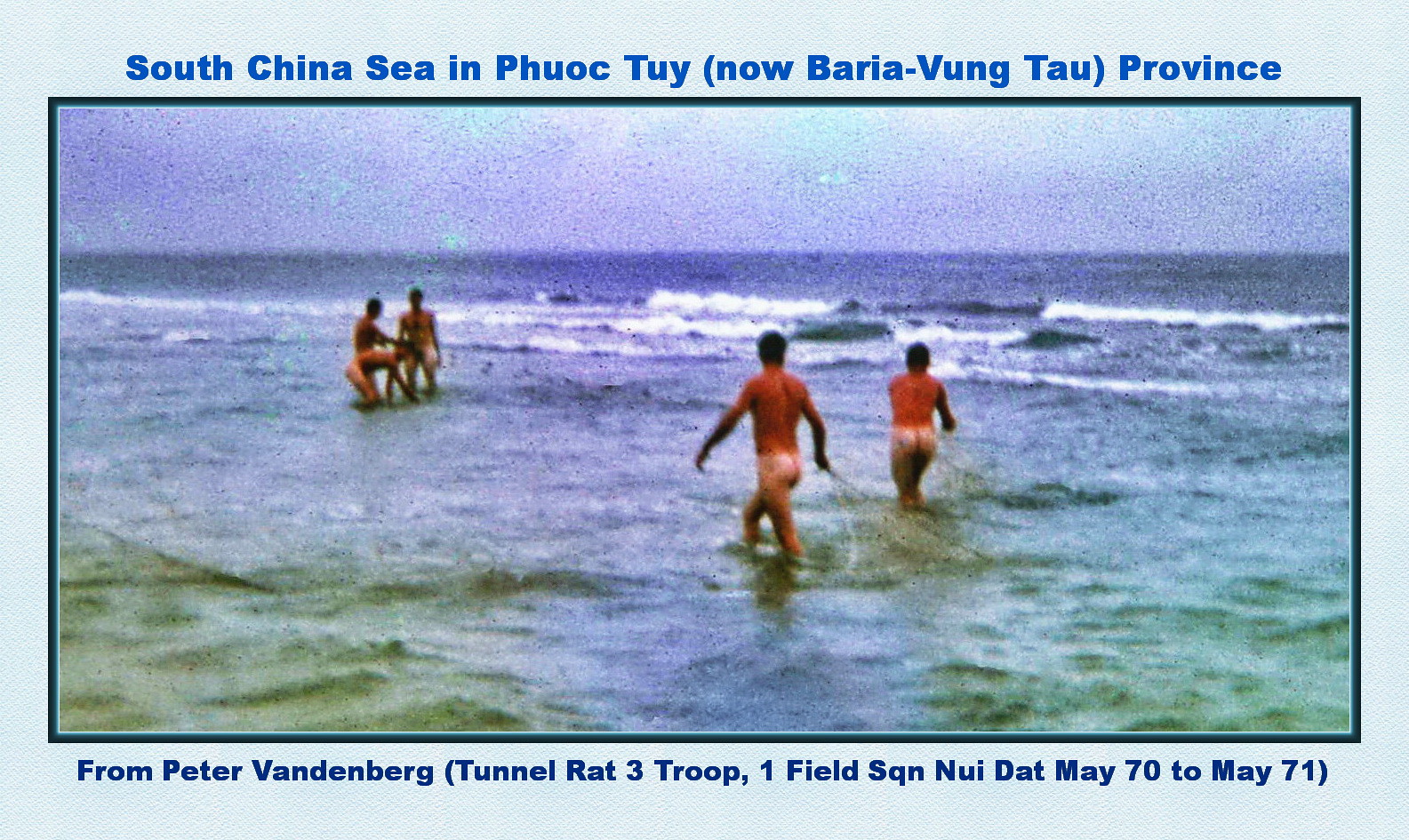This wide rectangular image, bordered in a light blue, textured frame, captures a group of five nude men in the South China Sea near Phuoc Thai, Ngao Ba Ria Vung Tau province. The sky above is a light blue with a purple tinge, transitioning into the blue-green sea marked by gentle waves on the horizon. The image, with a dark turquoise border inside the frame, shows two suntanned men in the foreground with their white bottoms visible, indicating their nudity. Further ahead, three more men are clustered together, seemingly engaged with something in the shallow waters. The caption in bright blue font at the top of the frame reads, "South China Sea in Phuoc Thai, Ngao Ba Ria Vung Tau province." Below, in dark blue font, it states, "From Peter Vandenberg, Tunnel Rat Three Troop, One Field SQN, Nui Dat, May 70 to May 71." This vintage photo captures a moment from the past, possibly during a break or leisure time.